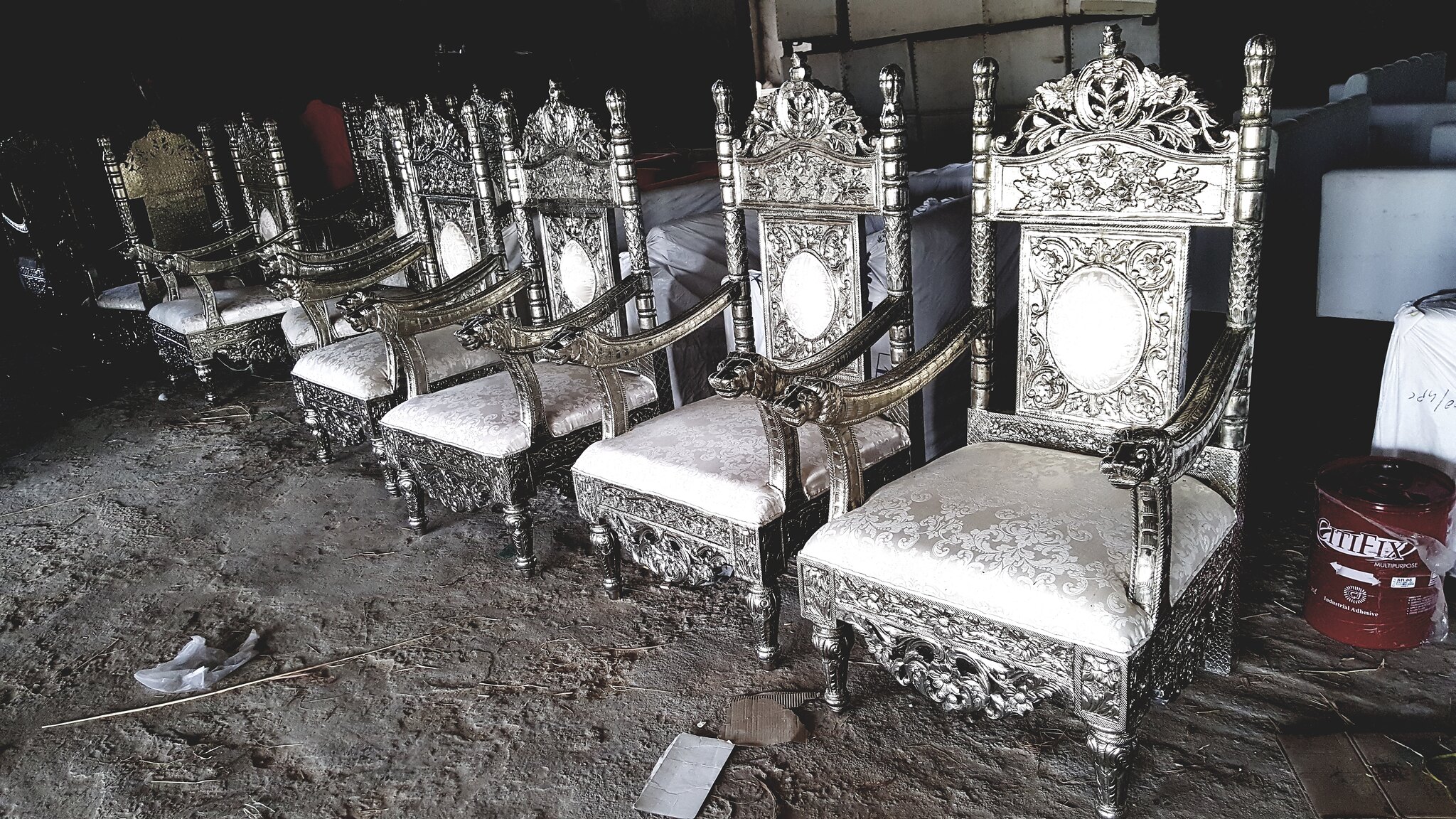The photograph appears to be taken indoors, possibly in a barn or a storage unit, where the upper left background is enveloped in darkness, creating a stark contrast with the more illuminated section of the image. Dominating the scene slightly right of center is a massive stone wall constructed from round, rectangular bricks held together by black mortar. The right side of the wall fades into the darkness again, creating a gradient of light to dark. Spanning the bottom half of the photo, from left to right, is a brownish dirt floor, dotted with visible footprints suggesting recent human activity.

The primary subjects of the photograph are seven identical and intricately designed chairs, evenly spaced across the dirt floor. Each chair features a white pillowed seat cushion and a back adorned with delicate and ornate floral patterns, likely crafted from some form of metal, perhaps silver. This silvery design, coupled with the regal aesthetic of the chairs, evokes a medieval, royal ambiance. The chairs, which also have embroidery on the seat cushions, exhibit a high degree of craftsmanship characteristic of artifacts or heirlooms, hinting they might be part of a restoration project or an exhibit of historical items.

Toward the right side of the image, approximately three-quarters up from the bottom, there is a bucket whose color is ambiguous due to the lighting—appearing either red or black—with unreadable white text on it. Scattered around the chairs are various objects, including boxes and other indistinct items, contributing to the impression of the setting being a storage space. The visual emphasis remains firmly on the row of elaborate, throne-like chairs, which stand out against the otherwise utilitarian backdrop.